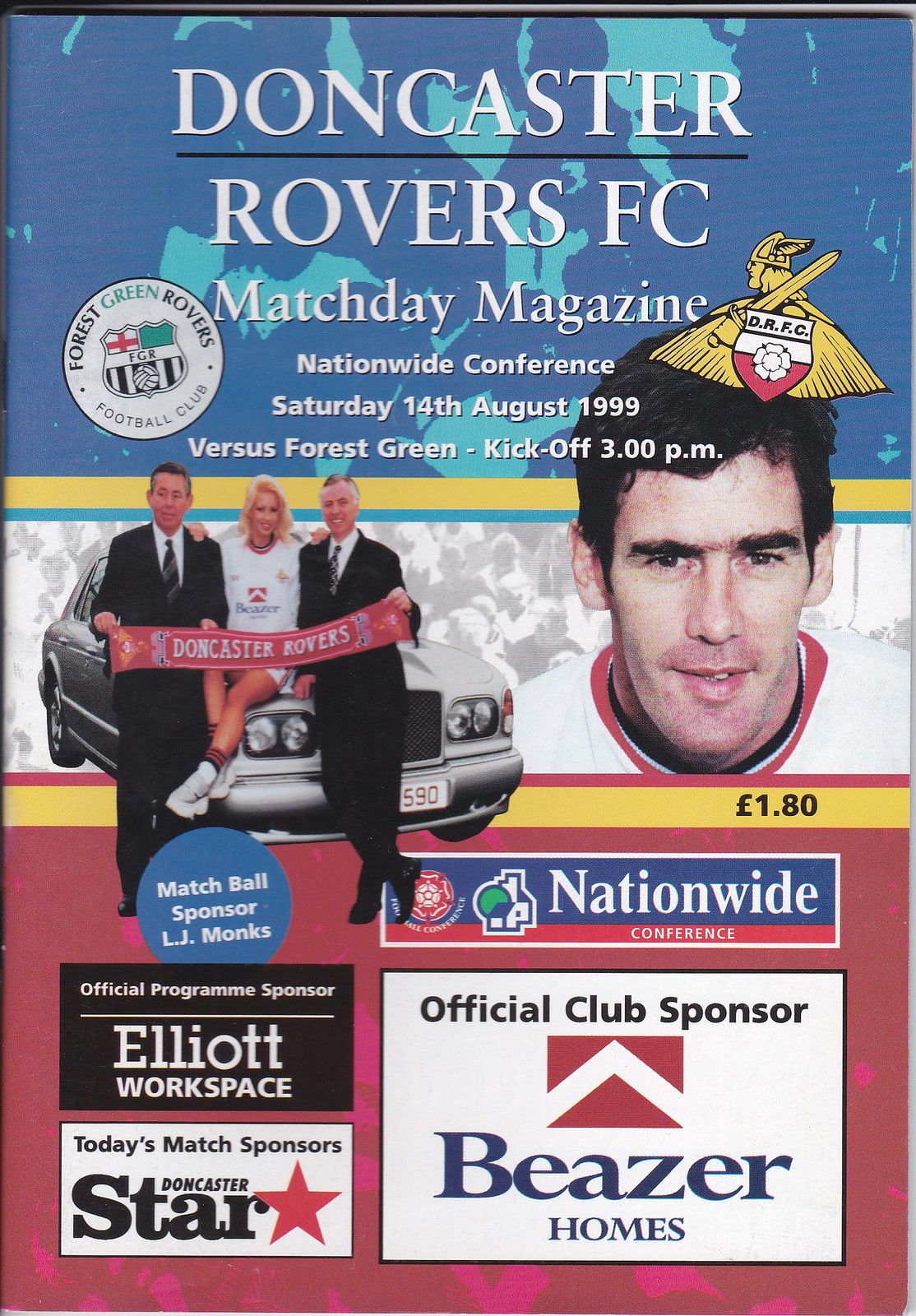This is a detailed photograph of the cover of a Doncaster Rovers FC Match Day Magazine from the Nationwide Conference, dated Saturday, August 14th, 1999, for a match against Forest Green, with a kickoff at 3 p.m. At the top, the magazine features the white text "Doncaster Rovers FC Match Day Magazine nationwide conference Saturday 14th, August 1999 versus Forest Green kickoff 3 p.m." Flanking this text are the team logos: the Forest Green Rovers Football Club emblem on the left and the Doncaster Rovers Viking logo on the right.

Below this heading, the left side of the cover showcases a photograph featuring a silver car. Two men in business suits are holding up a red banner that reads "Doncaster Rovers," with a blonde woman in a white shirt, shorts, and sneakers seated on the car's hood. To the right of this image is a close-up of a soccer player's face.

Additional text at the bottom of the cover lists the sponsors: "match ball sponsor LJ Monks," "nationwide conference official club sponsor Beezer Homes," "official program sponsor Elliott Workspace," and "today's match sponsors Doncaster Star."